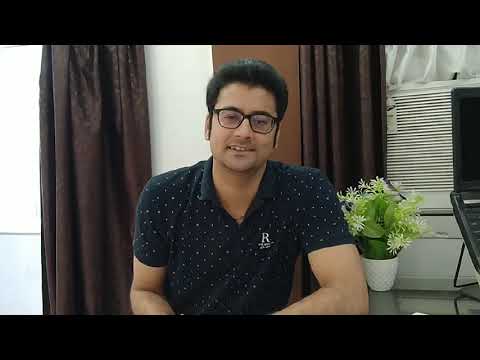The image features a man with light brown skin, dark hair combed backwards, and black square eyeglasses, seated at a table and smiling toward the camera. He is wearing a blue polo shirt with white specks, a collar, and an "R" insignia on the left chest. The background consists of brown curtains framing an open window that allows light to stream in. To his right, there is a wall-mounted air conditioning unit. On the table, the man's elbows are bent and resting, next to a white flower pot with green leaves and white flowers, likely artificial. Also on the table is a black object with legs, possibly an electronic device or stand, positioned towards the edge of the frame. The setting appears to possibly be a hotel room or a similar domestic interior. The photo is bordered at the top and bottom by black horizontal bands.